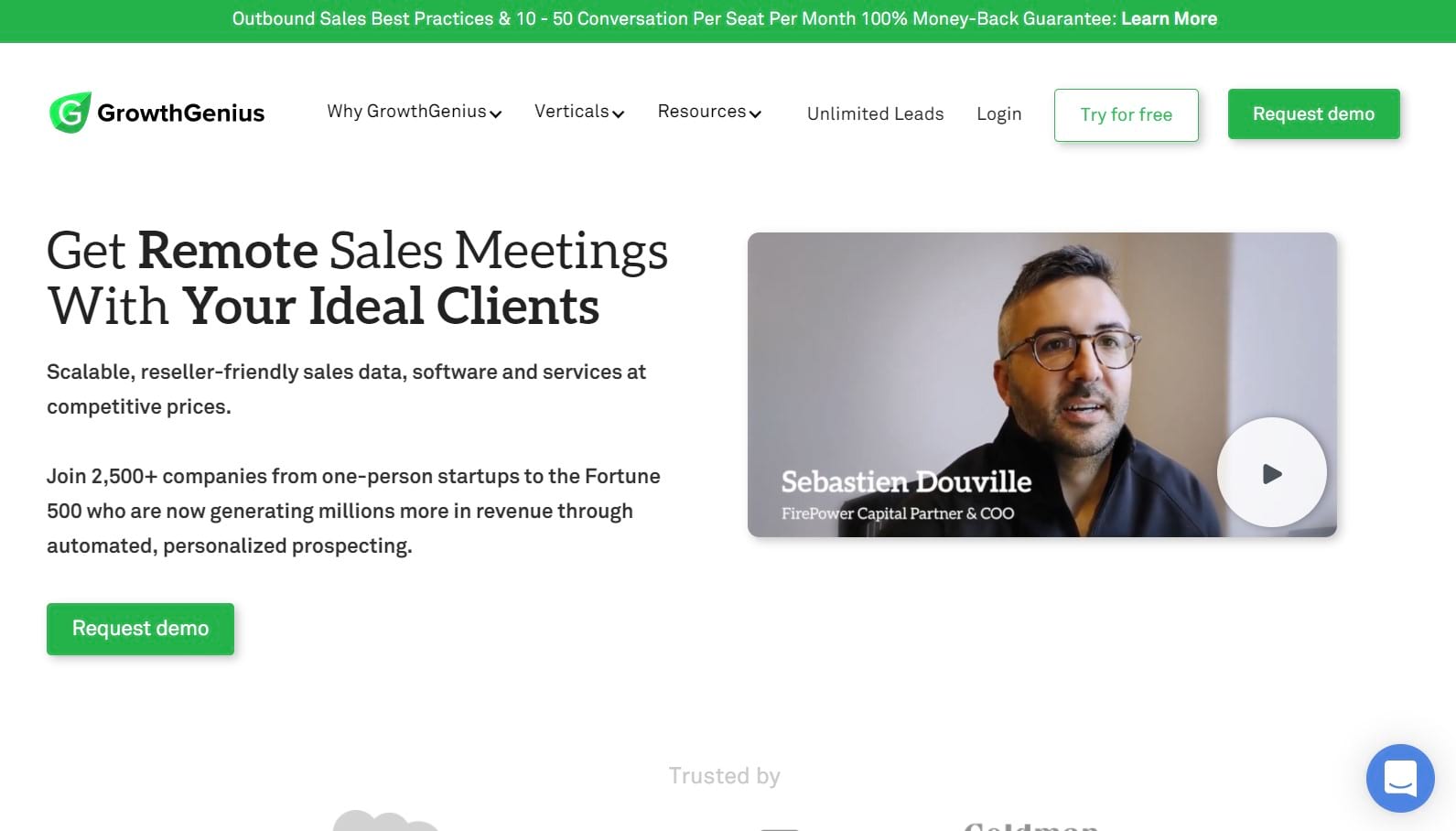**Caption for Image:**

The depicted website focuses on outbound sales best practices and personalized prospecting techniques. The primary headline reads, "Outbound Sales Best Practices: From 10 to 50 Conversations Per Seat Per Month," emphasizing a 100% money-back guarantee. The site promises insights and guidance to achieve growth, branding itself as "Growth Genius." 

Key sections of the website include:
- Why Growth Genius
- Verticals
- Resources
- Unlimited Leads
- Login
- Try for Free
- Request Demo

There is an emphasis on securing remote sales meetings with ideal clients, offering scalable, reseller-friendly sales data software services at competitive prices. The platform proudly serves over 2,500 companies, ranging from one-person startups to Fortune 500 firms, helping them generate millions in additional revenue through automated, personalized prospecting. 

A prominent green button with white text invites users to "Request Demo." To the right, we see a testimonial from Sebastian Deauville, the Firepower Capital Partner and Co-COO. His profile is highlighted with a large, circular play button allowing users to watch a video. Sebastian is described as a fair-skinned male with short hair styled with the sides cut short, sporting a trimmed stubble beard and glasses.